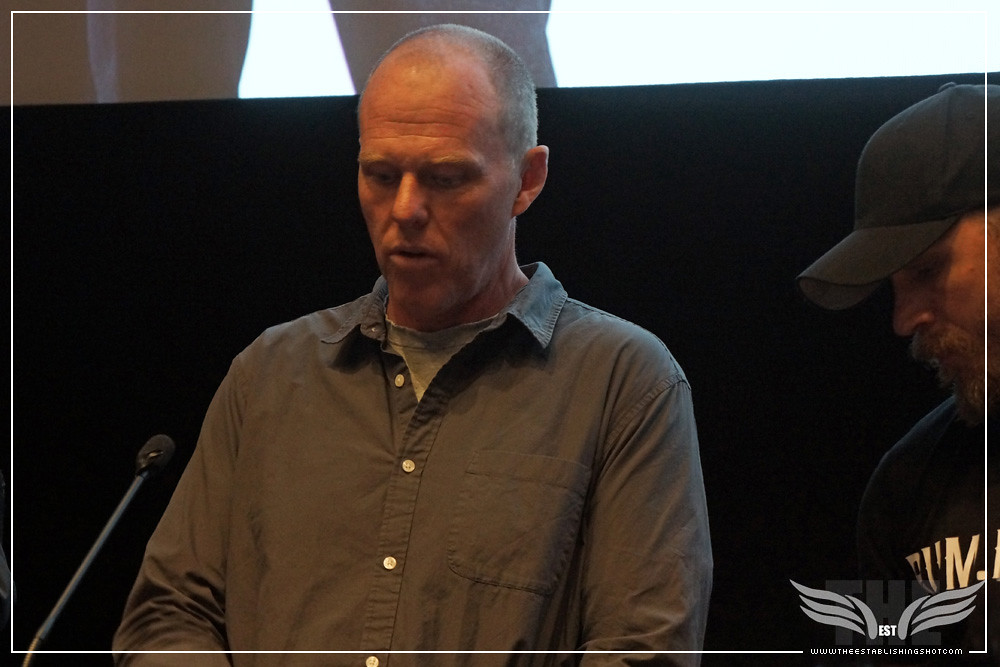The image captures director Brian Helgeland at what appears to be a speaking event. Helgeland is wearing a gray-green button-up shirt with a breast pocket, layered over a light gray t-shirt. He has thin, shaved hair and is looking down at something in front of him, possibly checking notes, while speaking into a black microphone positioned from the bottom left corner of the image. To Helgeland's right is another man, partially visible, wearing a black t-shirt and a black baseball cap, with a beard and mustache. The background is relatively dark with some light sources illuminating the subjects. In the bottom right corner, there is text that reads "www.theestablishment.com" and the watermark "EST".